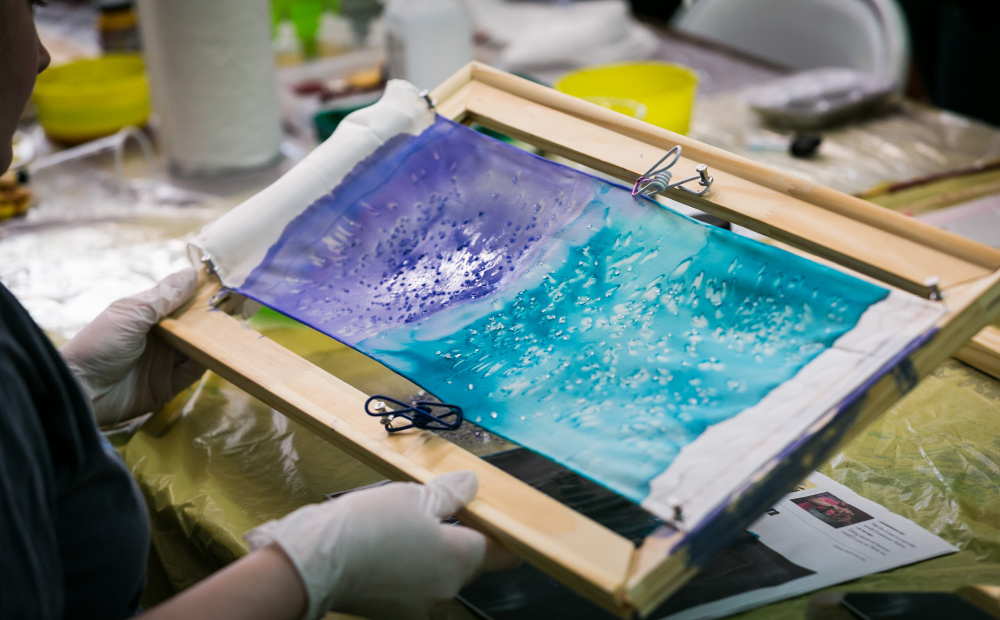This full-color photograph, taken indoors in Dover under artificial light, captures an artist engaged in a detailed painting project. The image is horizontally rectangular and features no distinct borders or background. Central to the photo are the artist's white rubber-gloved hands emerging from the lower left-hand corner, firmly gripping a brown wooden frame. This frame is equipped with paper clip-like attachments that stretch a white cloth canvas. The painting on the canvas features a striking gradient with purple hues on the left transitioning into a greenish-blue or teal color on the right, adorned with white speckles.

Surrounding the focused scene are various elements contributing to an artisanal ambiance. A yellow tablecloth beneath the canvas is partially visible along with a piece of paper that contains some writing. The blurred background reveals a cluttered workspace, featuring overturned clear plastic cups, yellow containers, assorted paints, and the barely visible top of a chair in the upper right corner. This photograph not only showcases the vibrant and intricate art being created but also encapsulates the dynamic environment of the artist's studio.